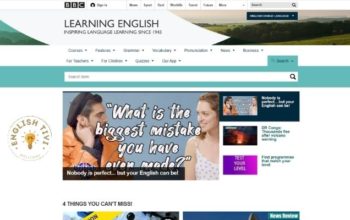This image depicts a somewhat blurry front page of the BBC website. At the top, despite the blur, there appear to be options like "Sign Up," "Music," and a "Search Bar," though the exact labels are unclear. Below this header section, there's a banner that reads, "Learning English: Pushing Language Learning Since 1941." The page is populated with additional sections including vocabulary and punctuation, though the other categories are indiscernible due to the image quality.

Further down, there is another search bar followed by a prominent video featured on the front page. The video titled "What is the Biggest Mistake You Have Ever Made?" features a man wearing a beret and a woman in a tank top, looking at each other. A caption below suggests a humorous take on the man's beret with the phrase, "Nobody is Perfect. Test Your English."

On the left-hand side of the screen, there's a small circular icon with the label "English TV" accompanied by an image of a light bulb, perhaps indicating educational content or innovative learning ideas. Lastly, on the right-hand side of the page, there seem to be a lineup of favorite videos, with the first being the previously mentioned "What is the Biggest Mistake You Have Ever Made?" Another video appears to be related to space, while a third one shows a predominantly purple and white screen, though the details of these videos are not legible.